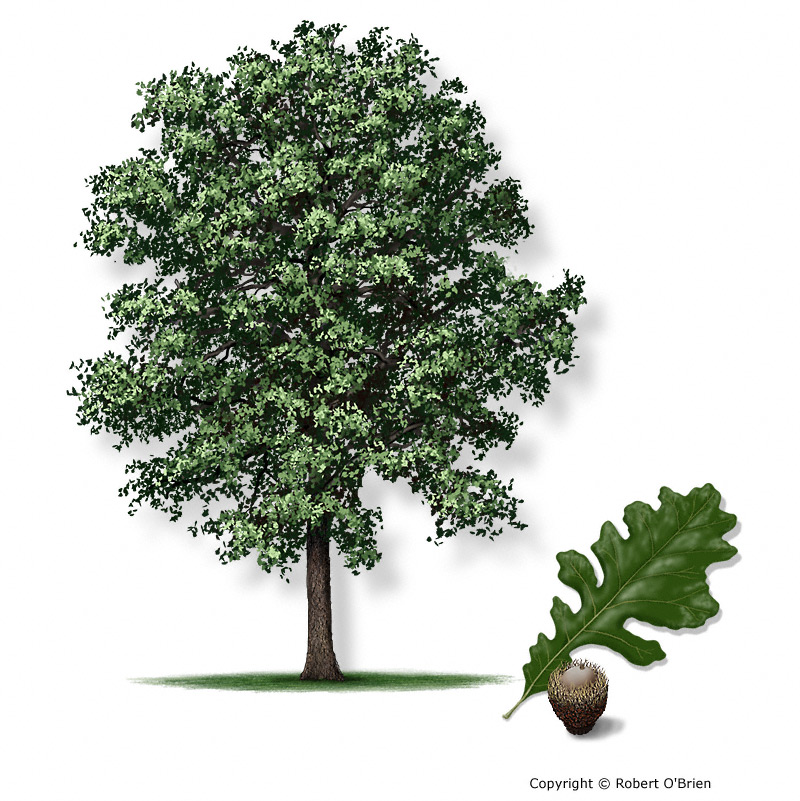This detailed botanical illustration features a tree, its leaf, and its nut, all meticulously depicted against a pristine white background. At the center is the tree, showcasing a brown trunk encircled by verdant ground cover and lush green foliage. The tree's canopy forms an elegant oval shape. Positioned on the lower right is a close-up of a leaf, characterized by its irregular edges. The leaf displays a rich dark green hue with light green highlights, while prominent light green veins run through its center, ending at the stem located at the bottom center. In the forefront lies a nut resembling an acorn; its base is a deep brown, topped with a light brown dome capped by a tiny stem. The illustration is credited to Robert O'Brien, whose name is inscribed in small black text at the bottom.